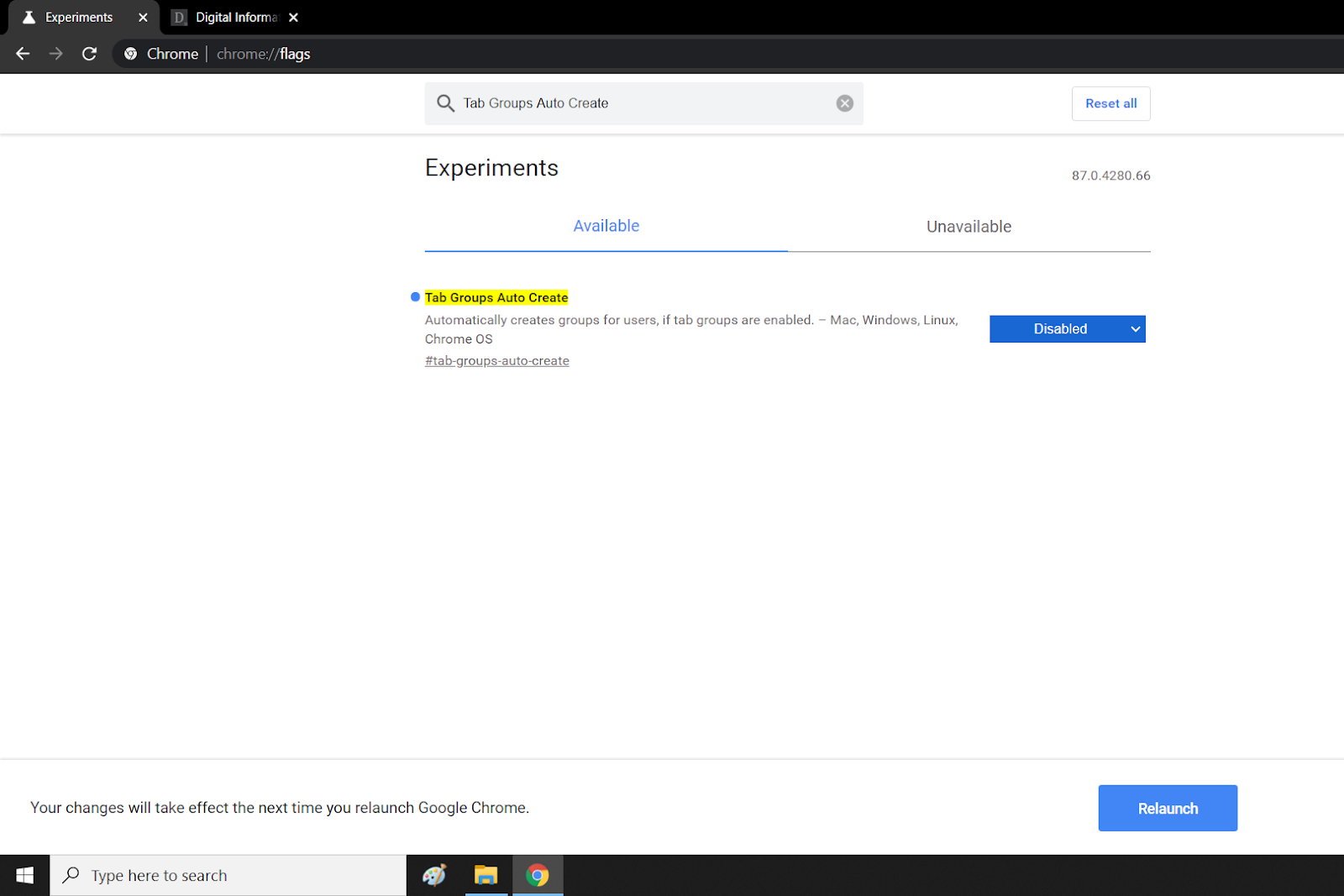The image depicts a Chrome browser window showcasing the experimental feature settings page, indicated by the URL "chrome://flags" in the address bar. At the top of the page, there are standard browser navigation elements: a back button, a refresh button, and the address bar itself. The page includes a search box in which the term "tab groups, auto create" is entered.

Beneath the search box, the page lists various experimental features. One such feature is labeled "Experiment 87.0.4280.66." The page is divided into sections marked "Available" and "Unavailable," with the "Available" section highlighted in blue, indicated by an underline and a blue circle.

The focused feature, "Tab Groups Auto Create," is prominently highlighted in yellow. Below this, it is described as a function that automatically creates tab groups for users if the tab groups feature is enabled. This feature is applicable across multiple operating systems, including Mac, Windows, Linux, and Chrome OS. Adjacent to this description, there is a blue button with a drop-down icon labeled "Disabled," indicating the current status of this experimental feature. Additionally, there is a "Reset all" button at the top of the page to revert any changes made to the experimental settings.